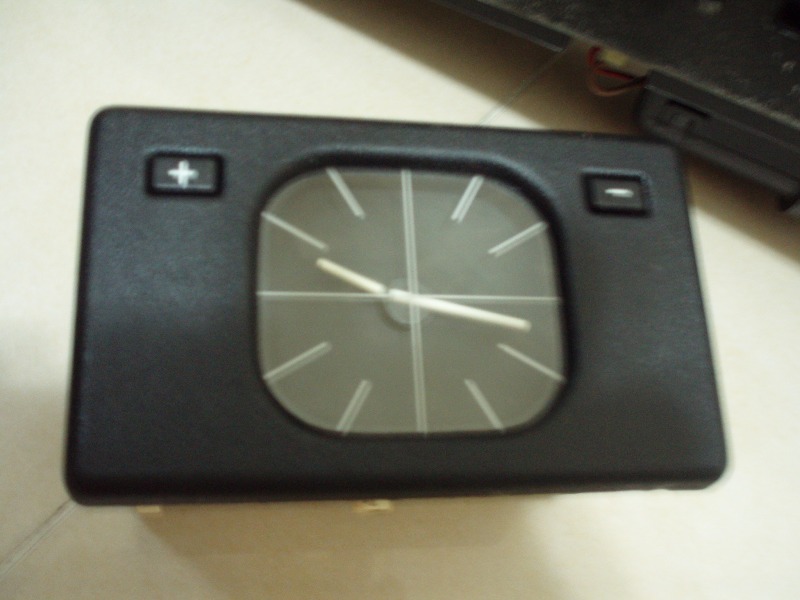The image depicts a slightly out-of-focus photograph featuring a small, travel digital clock, centered on a white background, likely a table. The clock is housed within a simple black rectangular plastic casing. Its face, a rounded oblong shape, displays time without traditional numbers, using white dashes in place of hour markers, and has two white clock hands. On the top left corner of the clock, there is a small button marked with a plus symbol, while on the top right corner, there's a matching button with a minus symbol. Both buttons are white. The photograph's blurriness suggests it was taken hastily with a regular camera. Additionally, in the top right corner of the image, there is an indistinct, dark grey object, possibly a scuffed metallic file. The clock shows the time as approximately 10:18.